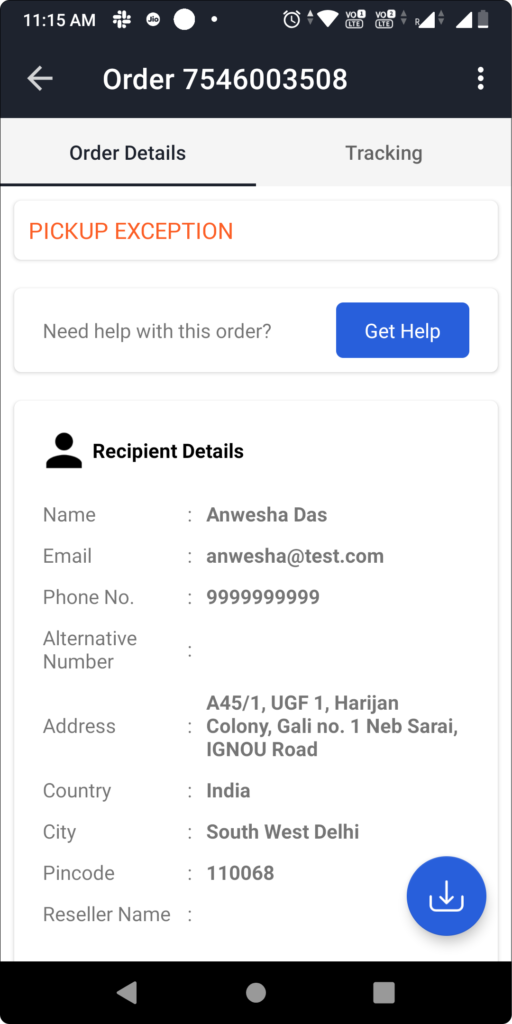This image is a detailed screenshot of a mobile application interface. The top of the screen features a dark gray header with white icons on the left and right corners. On the left, there is a white arrow pointing to the left, while the center displays the text “Order 7546003508” in white. On the far right, three vertically stacked white dots are visible.

Beneath the header is the main body of the page, which starts with a light gray section underlining two buttons. The button on the left is labeled "Order Details" in bold black text and is underlined by a thin black line, indicating it is the selected or active tab. The button on the right is labeled "Tracking" in dark gray text.

The primary content area consists of several white rectangular panes with rounded corners. The first pane, almost the width of the page but not very tall, contains orange text in all caps in the middle that reads "PICKUP EXCEPTION." Directly below this pane, another similar-sized pane holds smaller, centered light gray text on the left that says "Need Help With This Order," and to the right of this text is a blue button with rounded corners labeled "Get Help" in white text.

The final pane stretches to the bottom of the page and holds various recipient details. It begins with a black profile picture icon on the left, followed by bold black text "Recipient Details" on the right. Below this title, detailed rows of information are listed, with each row containing left-justified light gray text indicating the category, followed by a colon and the corresponding bolded dark gray information.